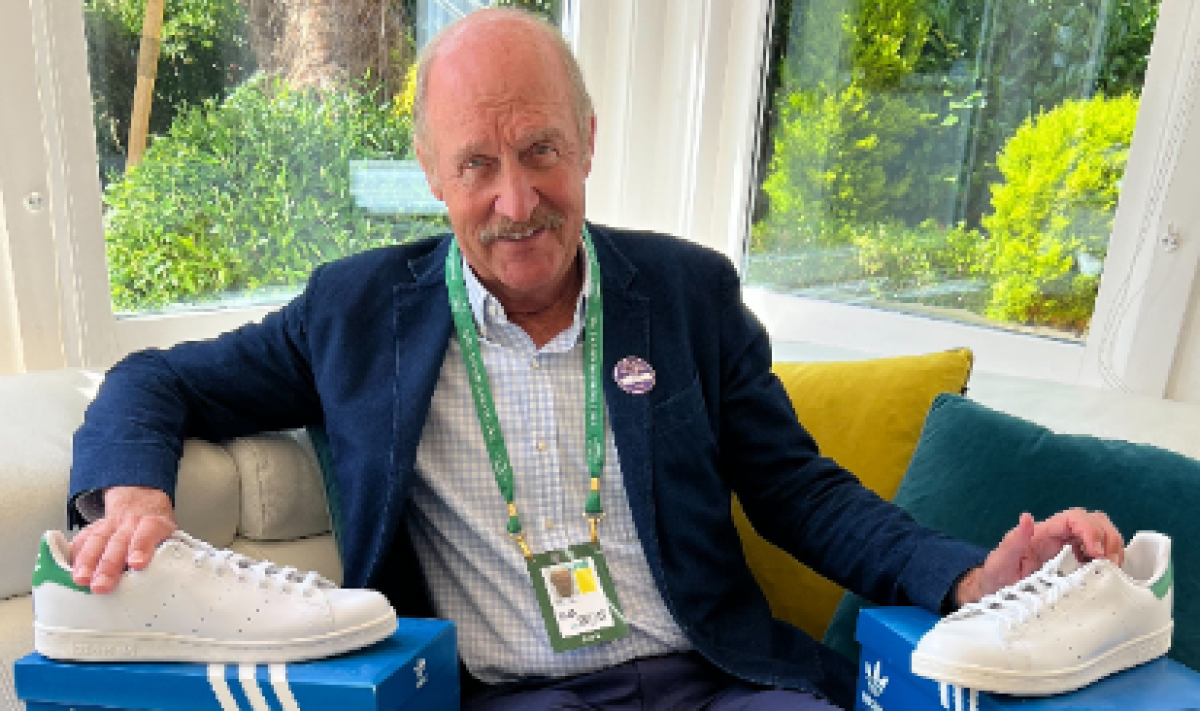In a well-lit bay window space, an older Caucasian man, likely in his 60s or early 70s, sits smiling warmly. He sports a well-manicured mustache and has thinning hair at the sides of his head, while appearing bald on top. He wears a green lanyard around his neck, attached to a name tag, suggesting he might be at a conference. Dressed in a navy blue blazer adorned with a circular lapel button and a white button-up shirt with a blue checkered pattern, he exudes a casual yet sharp look.

Seated on a smooth white couch with a yellow-green pillow to his left, the man has one hand resting on each of the white Adidas sneakers in front of him. The sneakers, featuring a green accent around the heel, sit atop two blue Adidas boxes. With his head slightly tilted down, he directs his smile towards the camera, his front teeth showing. Behind him, angled windows offer a view of lush trees and bushes, adding to the serene ambiance of the scene. The man’s sneakers, meticulously laced and brand new, suggest a recent purchase or perhaps a prized possession.